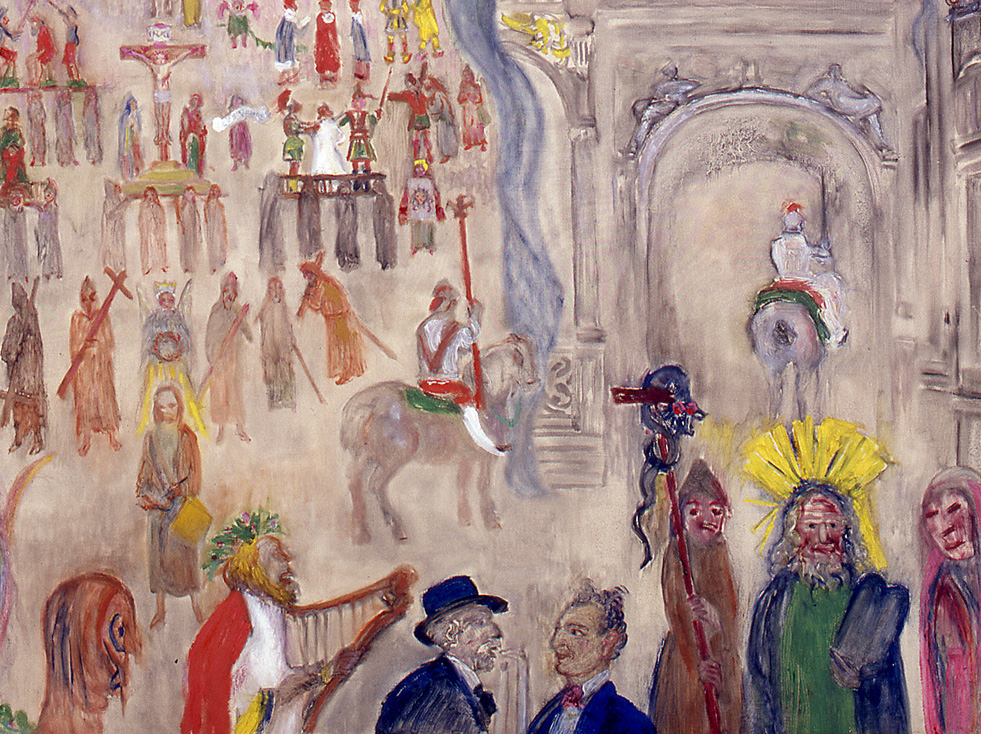This painting features a complex and detailed scene set against a gray background, filling a wide vertical rectangular canvas. The artwork depicts a chaotic and somber parade-like procession with a contrast of vibrant colors and drab tones, emphasizing the gravity of the scene. In the foreground, there is a person adorned with a bright yellow headdress, standing beside another individual in brown robes who carries a cross topped with a skull. Central to the image is a man on a horse, dressed in a costume with a brown sash, holding a staff or sword. Another notable figure is a harp player, crowned with greenery, sporting shaggy hair, a beard, and a red cape over white garments. A woman, clad in a long blue and yellow dress, carries a wreath, while other participants don long tunics and carry crosses. In the background, smaller, less detailed figures are drawn in light reds. These include a depiction of Jesus nailed to the cross, a woman held by two soldiers, and numerous gray-cloaked individuals. An architectural element—a gray, arched castle opening—frames some of these figures, including a soldier with a sword. A woman in a brown cloak, holding a staff topped with a gray skull, appears in the bottom right alongside a man with a yellow feathered arched hat, dressed in a green and blue cloak, and another woman in a red cloak marked by red blood on her face. The entire scene exudes a sense of horror and sorrow, capturing a historical and emotional narrative through a blend of realism and abstract elements.